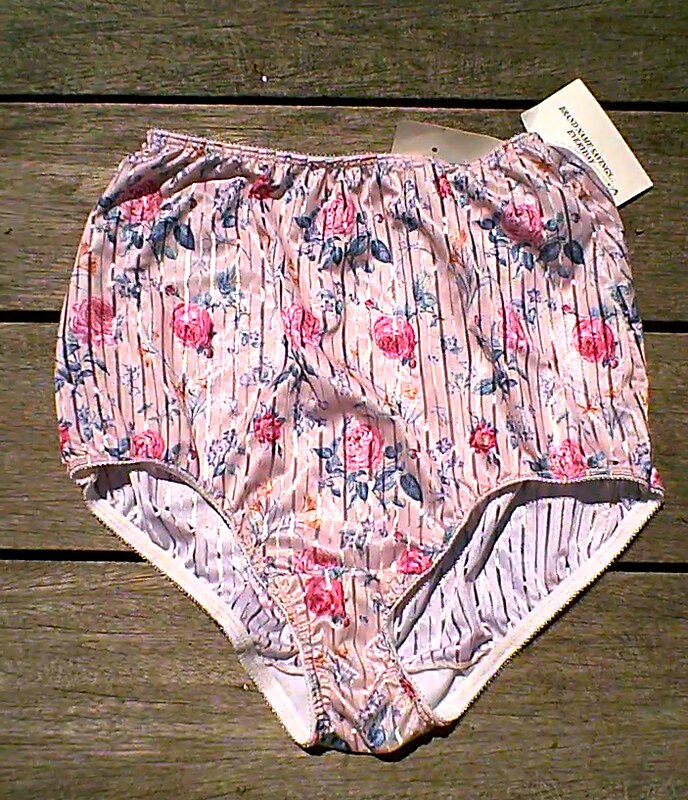In the center of the photo, which is set against a dark brown, wooden backdrop suggestive of a picnic table or deck, lies a pair of pink women's underwear. The wooden surface features visible planks with black gaps between them. The underwear, characterized by a traditional, high-waist style, is adorned with vertical golden stripes and a vibrant floral design comprising red bulb-like flowers with blue stems and greenery. Two white tags are attached to the back of the underwear; however, their black text is not legible.